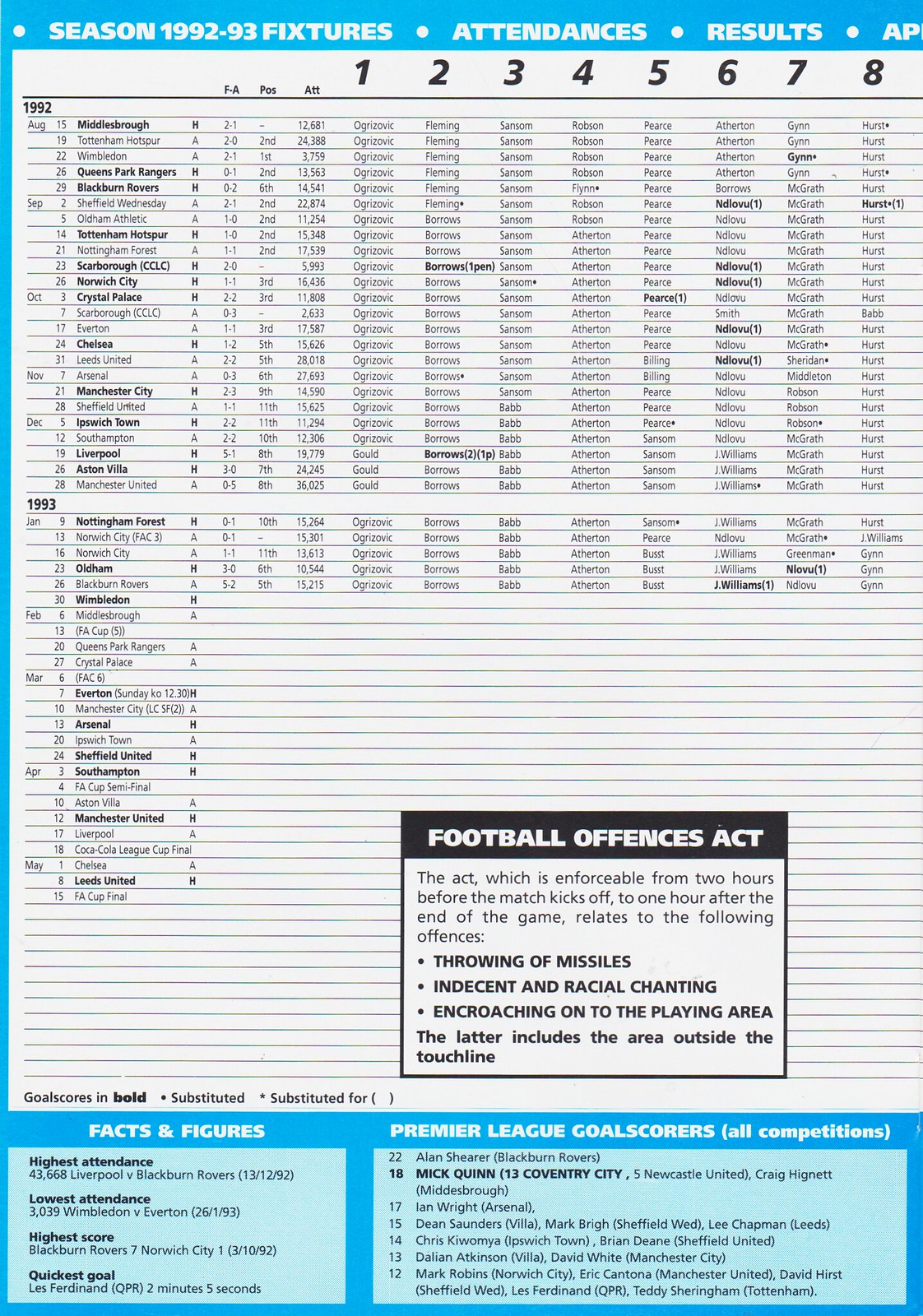The image is a detailed and elongated vertical, rectangular soccer schedule from the 1992-93 season. It features a bright blue inner border framing a white section, resembling a lined sheet of paper. At the top, against the blue background, it reads: "Season 1992-93 Fixtures, Attendances, Results, and AP." The schedule comprehensively lists every team vertically with horizontal details such as positions, scores, and attendances. 

Beneath the dense chart, which spans the years 1992 and 1993, there are two key sections. The first is a small black rectangle providing information about the "Football Offenses Act," enforcing regulations from two hours before to one hour after matches, covering offenses like missile throwing, indecent and racial chanting, and player area encroachment. 

At the very bottom, within light blue rectangles, are additional statistics and data, including "facts and figures" on one side and a list of "Premier League goal scorers" on the other.